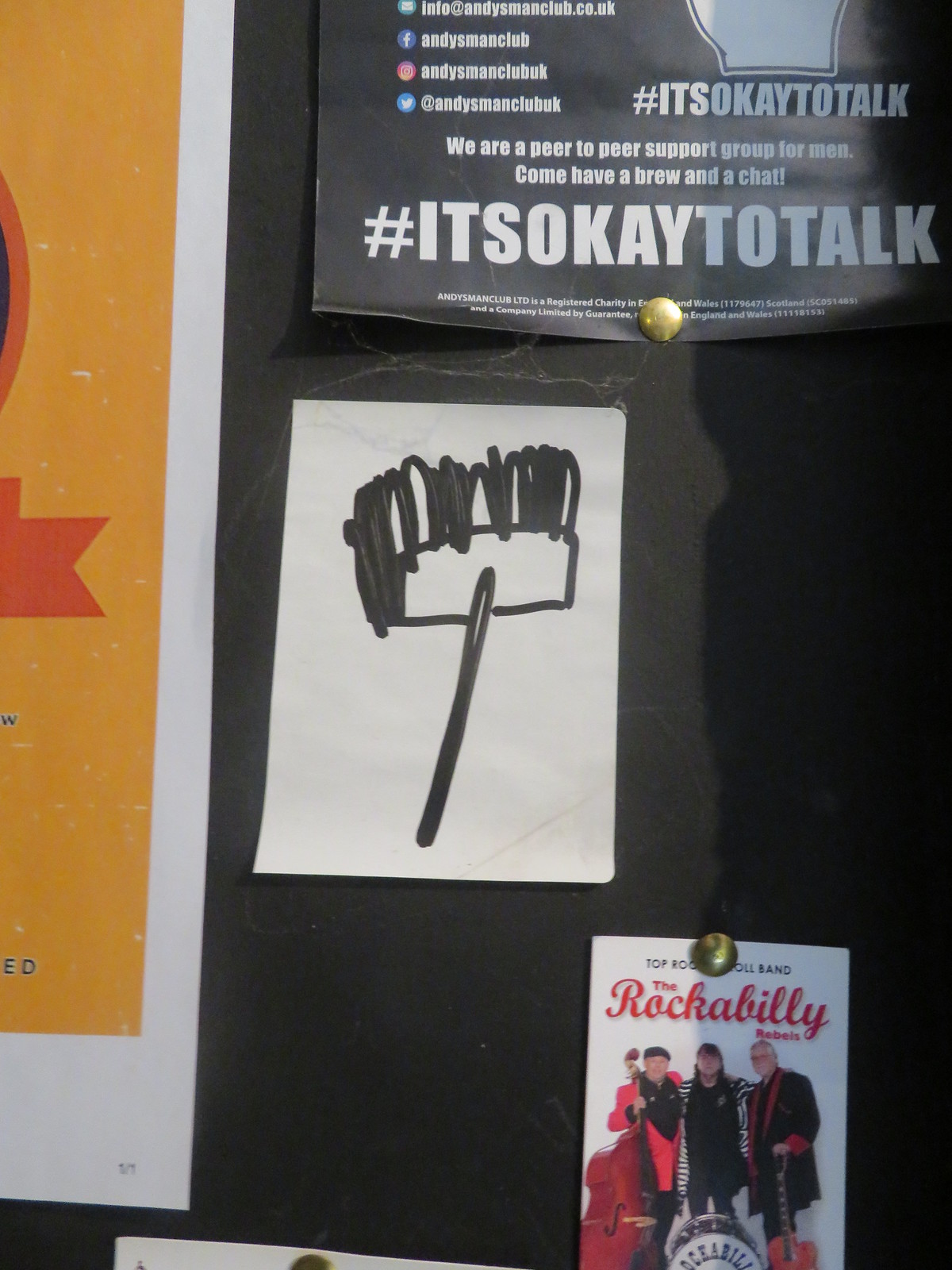This image depicts a close-up of a bulletin board commonly found in schools or dorm hallways, covered in black paper. Prominently displayed in the top section is a flyer pinned at the bottom with the message, "It's okay to talk." The flyer belongs to Andy's Man Club, a peer-to-peer support group for men, encouraging them to join for a chat over a brew. Social media links for Andy's Man Club on Facebook, Instagram, and Twitter are also visible. Below this, there's a white piece of paper featuring a quickly drawn sketch of a broom or bristle brush, and beneath it, a flyer for a Rockabilly concert. The Rockabilly Rebels poster, pinned with a gold thumbtack, shows an image of three older band members holding an upright bass, guitar, and a bass drum. Off to the left, there's a partial poster with a gold center framed in white, featuring some red and orange shapes.